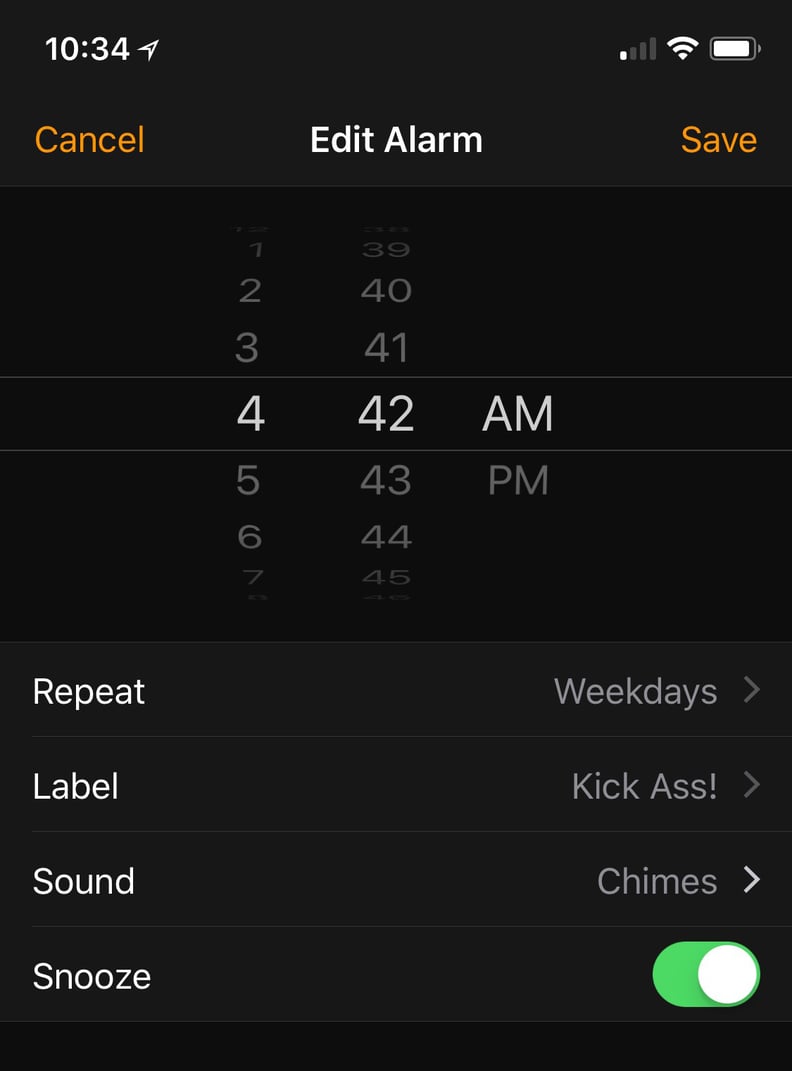The tall rectangular image, evidently a screenshot from a smartphone, reveals the "Edit Alarm" interface commonly found on mobile devices. 

At the top is a dark gray status bar featuring key phone statistics. From left to right, it shows the time "10:34" in white, followed by a white angled triangle pointing to the upper right, similar to the positioning of notifications. To the far right, the status bar displays a weak Wi-Fi signal with just the smallest bar highlighted in white, the Wi-Fi symbol itself in white, and a near-full battery icon.

Below this status bar, the alarm editing interface is organized with "Cancel" in orange on the left, "Edit Alarm" in white at the center, and "Save" in orange on the right. Directly underneath these options is a black background section containing a dual-column number roller. The left column shows a sequence of hours from 1 to 7, with the numbers 1 and 7 slightly hidden at the top and bottom edges, indicating scrollability. The right column displays minutes from 39 to 45, similarly arranged. To the right of the minute column, the options "AM" and "PM" are listed in large white letters and smaller gray letters, respectively, with "AM" highlighted. At the intersection of the columns, "4:42 AM" is prominently displayed in white, denoting the selected wake-up time. 

Further down, a gray box outlines additional alarm settings. "Repeat" is indicated in white letters on the left and "Weekdays" in gray letters on the right, accompanied by a right-pointing gray arrow. Below this, under the label "Label," the phrase "Kick ass!" is displayed in gray, followed by another right-pointing gray arrow. A faint gray line separates these settings from the next: "Sound" is written in white on the left, while "Chimes" with a white arrow pointing right appears on the right. Directly beneath this, the word "Snooze" is in white, and a green toggle switch shows it is enabled, the white circle positioned to the far right within an oval green slider.

At the bottom of the image, a long, thin black bar completes the interface view. This comprehensive screenshot exemplifies the detailed settings available when configuring an alarm on a smartphone.